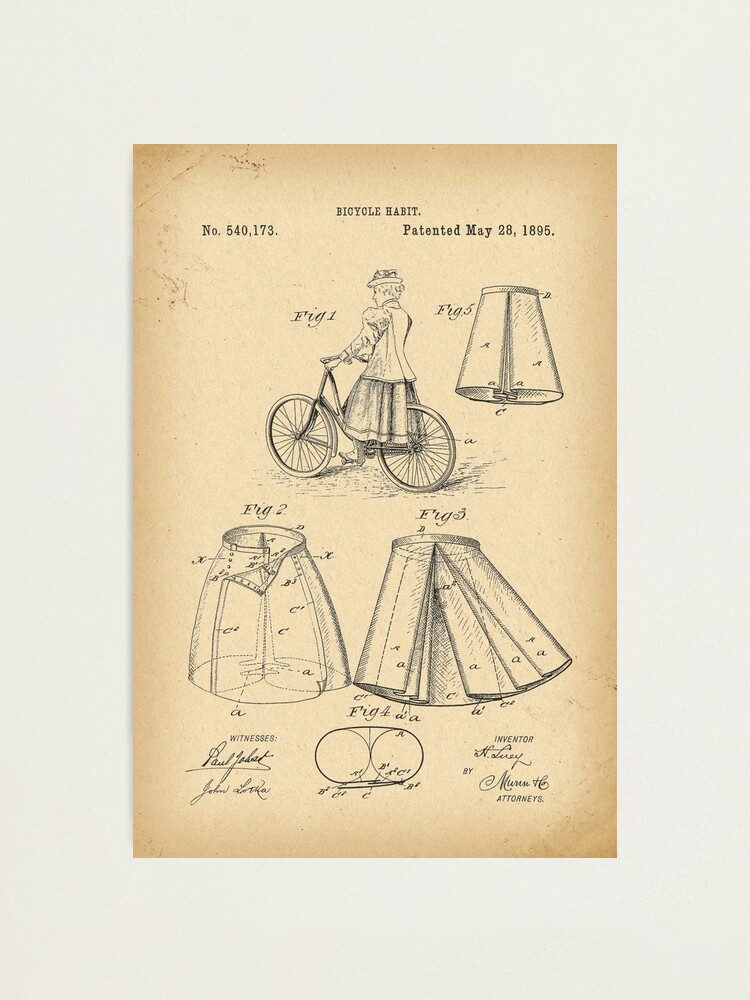The image depicts an aged tan piece of paper against a light gray background, bearing the patent number 540,173 for a "Bicycle Habit," patented on May 28, 1895. The document, designed like an old art print, features intricate black line drawings and text. It's numbered "N.O. 540173" and titled "Bicycle Habit." The primary illustration, labeled "Figure 1," shows a woman riding a bicycle while wearing a skirt. "Figure 2" illustrates the unique function of the skirt: it splits and drapes over the rear tire, preventing it from getting caught in the bicycle's mechanism. The skirt essentially acts as a protective, cone-shaped covering that maintains its form while enabling women to ride bicycles comfortably. The paper itself appears light brown with darker, aged edges, enhancing its historical essence.